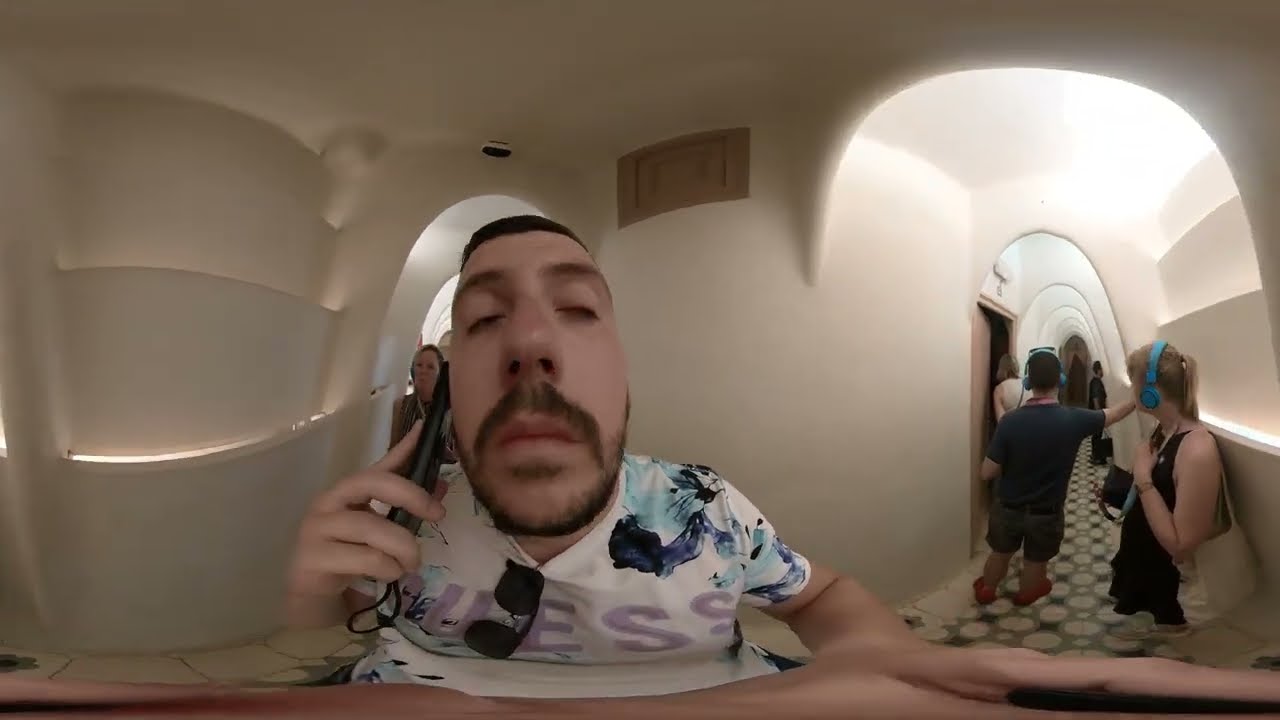The image is a color, landscape-oriented photograph that appears to be a distorted panoramic composition made up of three different shots of the same setting, creating a surreal and stretched effect. In the center of the image, a young Caucasian man, possibly in his mid to late 20s, is facing the viewer. He wears a white t-shirt adorned with blue, black, and purple prints on the shoulders and the word "GUESS" in purple across the chest. His dark hair and facial hair, including a bulbous nose and dark eyebrows, stand out. He holds a cell phone with a strap to his right ear using his right hand, while his sunglasses dangle from the neck of his shirt. His eyes are closed, and his head is slightly tilted back, almost revealing the inside of his nostrils. 

To his right, a woman in a sleeveless black outfit with a cream colored purse over her left shoulder walks through a white arched doorway that leads into a hallway with three layers of illuminated white walls. Behind her, another arched hallway can be seen with several people, some wearing headsets, all faced away from the viewer. One man in dark clothing, including dark shorts and possible red shoes, leans against the wall with sunglasses perched on his head. Another woman appears to be opening a brown door to the left side of the image.

The left part of the panoramic photograph shows a recessed area in the hallway with upward-projecting lighting. Overall, the white walls are bright and clear, adding to the slightly unsettling yet photorealistic and representational style of the intricate panoramic image.